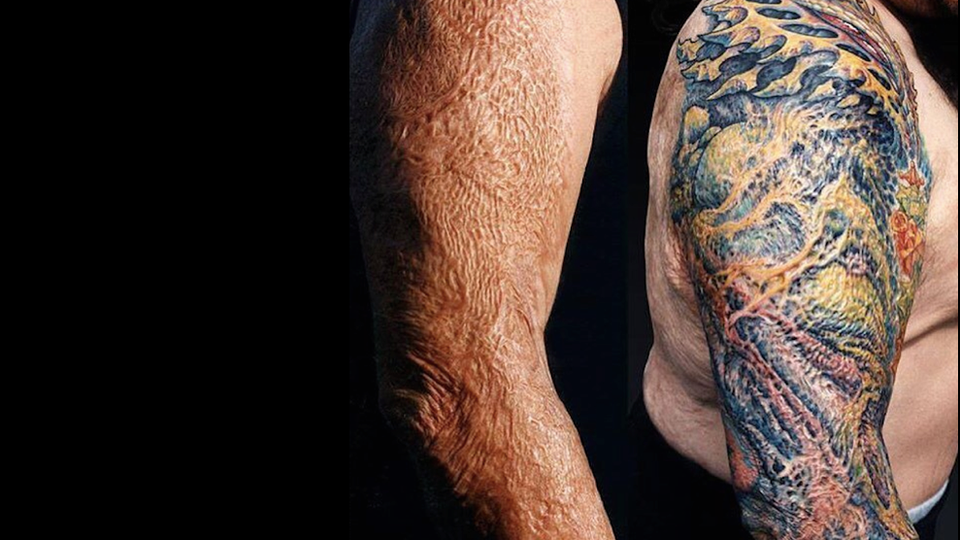The image features a stark black background, with the left side completely dark. At the center, an elderly person’s arm is prominently displayed from the shoulder down to just beneath the elbow, slightly bent as if the person is facing towards the right side. The skin on this arm appears not just aged but possibly burnt and heavily scarred, with a texture reminiscent of a cantaloupe, crisscrossing lines resembling veins. In front of this person stands another individual, similarly positioned sideways facing to the right. This second person's arm, slightly overweight, is covered in an elaborate, colorful tattoo featuring oranges, yellows, blues, and tans, suggesting an attempt to cover the scars. Despite the vivid colors, the tattoo pattern is difficult to discern clearly. This person is not wearing a shirt, further indicating a male body. The juxtaposition of the scarred and tattooed arms evokes the appearance of a 'before and after' scenario, possibly suggesting the process and result of tattooing over scars.